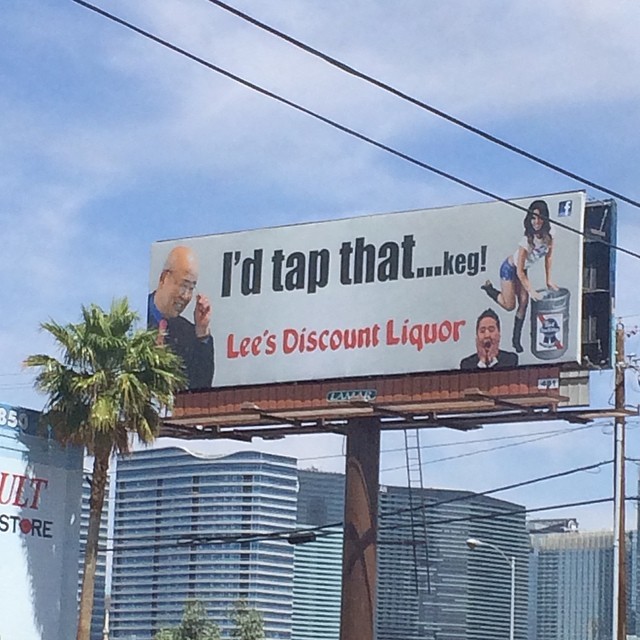This image captures a tall billboard from an angled perspective, standing prominently against a backdrop of urban structures and clear sky. The billboard, towering above a nearby building and a palm tree located in the bottom left corner, is mounted on a large, round, brown metal pole featuring a rectangular metal base inscribed with "Lamar."

The sky behind the billboard is a vibrant blue with very thin white clouds. Notably, power lines can be seen running from the top left corner diagonally towards the middle right, with additional power lines visible in the bottom right corner.

A small ladder is attached to the backside of the billboard, extending downwards towards the ground. The advertisement displayed on the billboard has a white background with bold, black text that reads, "I'd tap that… keg," accompanied by three dots.

On the left side of the billboard, there's an image of an Asian man looking down and smiling. The right side features a woman in short shorts and a tight T-shirt, striking a playful pose with her right leg kicked back and holding the top of a Pabst Blue Ribbon keg while smiling. Below her, towards the bottom right, there is a man with his hands on his face, depicted only from the torso up. The bottom of the billboard reads "Lee's Discount Liquor," completing the advertisement.